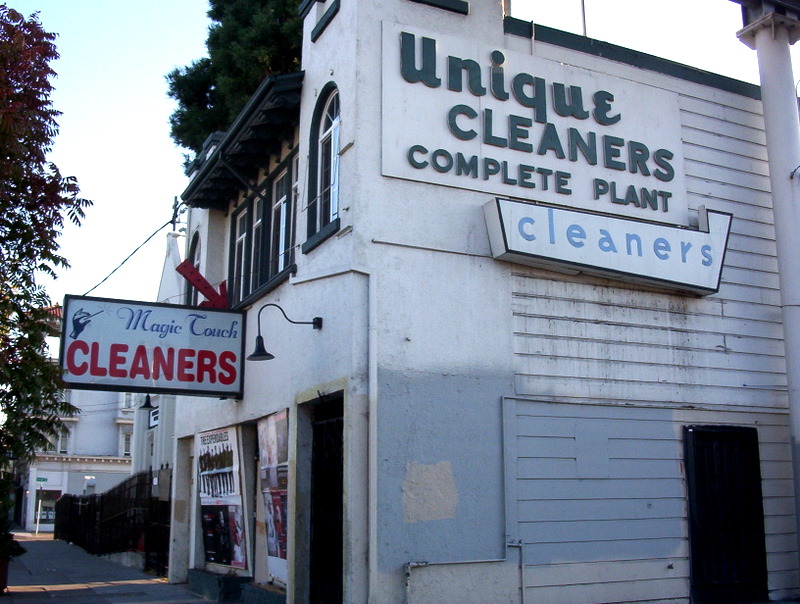This image depicts a two-story white stucco building in a small town, captured from an angled corner perspective. The front of the building features a protruding sign that reads "Magic Touch" in blue cursive font, accompanied by a red "Cleaners" text underneath, along with a small hand holding a wand illustration. Below the sign, there is an entrance door flanked by windows, some of which seem to be covered, with a lamp hanging above the door.

On the side of the building, prominently displayed at the top, is another sign stating "Unique Cleaners, Complete Plant," with the word "Cleaners" again in blue letters underneath. This side also showcases a mix of white paneling at the top and blue at the bottom, as well as a black doorway in the lower right-hand corner.

Surrounding the building, the scene includes some trees and foliage visible behind and to the left, contrasting with a clear white sky. To the left of the building, other structures can be seen in the distance, lining the sidewalk that runs along the front. The overall setting suggests early morning or evening, characterized by soft lighting.